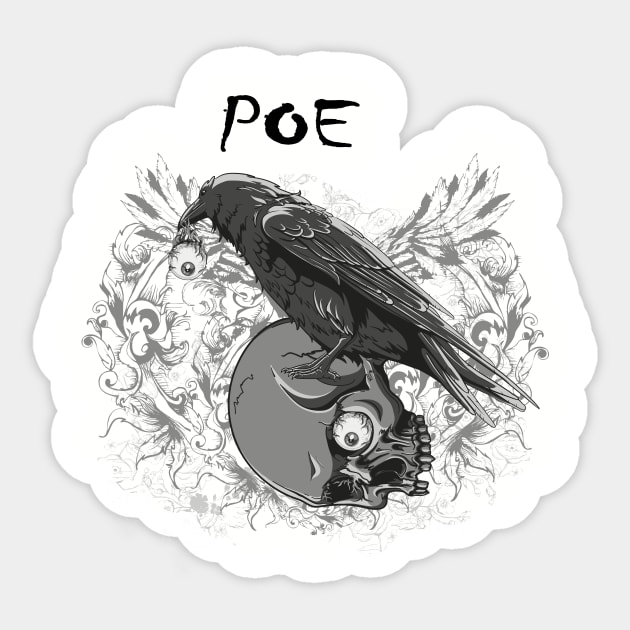This image showcases a highly detailed, artistic drawing or digital illustration set against a mild grey background. At the top center, the word "POE" is boldly inscribed in dark black ink, likely as a tribute to Edgar Allan Poe. The central focus is a striking black bird, presumably a crow, perched atop a human skull that is missing its lower jaw. The skull is oriented towards the viewer, with one eyeball still lodged in its socket, wide and bloodshot. The crow clutches the other eyeball in its beak, its optic nerve visibly dangling. The background surrounding the bird and skull features an array of feathers and squiggly lines, enhancing the intricate, tattoo-like aesthetic of the piece. This image captures a dark yet captivating scene, balanced between monochromatic tones of white, grey, and black.